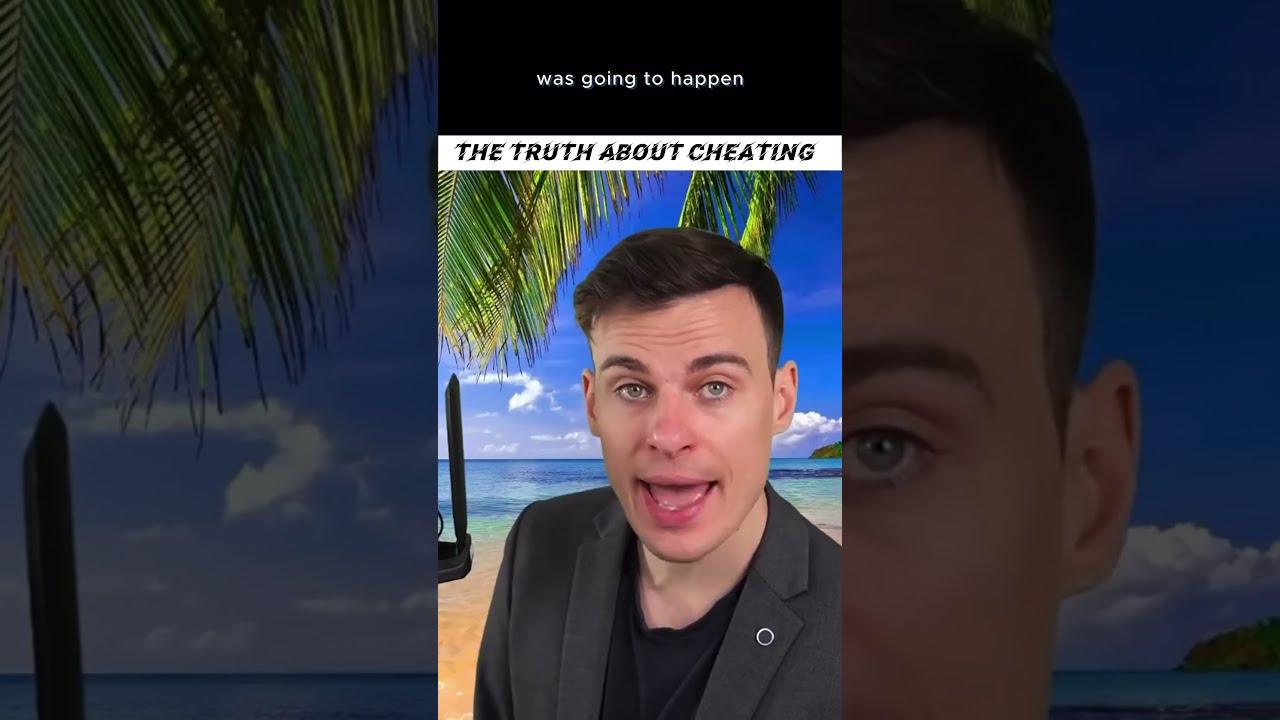The image features a young Caucasian gentleman with short brown hair, light-colored eyes, and fair skin. He appears to be speaking, with his mouth wide open, prominently showing his tongue, and we can see his bottom teeth partially. His eyebrows are raised, and there are wrinkles on his forehead, indicating an expression of surprise or emphasis. He is dressed in a gray dress jacket over a black crew-knit shirt, and a small circular silver lapel pin is visible on the jacket. 

The background is a digitally inserted tropical beach scene featuring palm trees, the ocean, and clouds, giving off a vibe of the Bahamas. The image employs a layered effect, with a smaller inset of the man in the center and an enlarged, cropped view of his face and eye extending into the right-hand third of the screen. Behind and around him, to the left and to the right, the tropical beach scene is visible.

At the top of the image, there is a black header with white text stating, "was going to happen." Below this is a white banner with angled black text reading, "the truth about cheating." The man's image has been clearly enlarged and used cleverly as an eye-catching background, emphasizing the intensity of his facial expression and the surrounding tropical aesthetic.